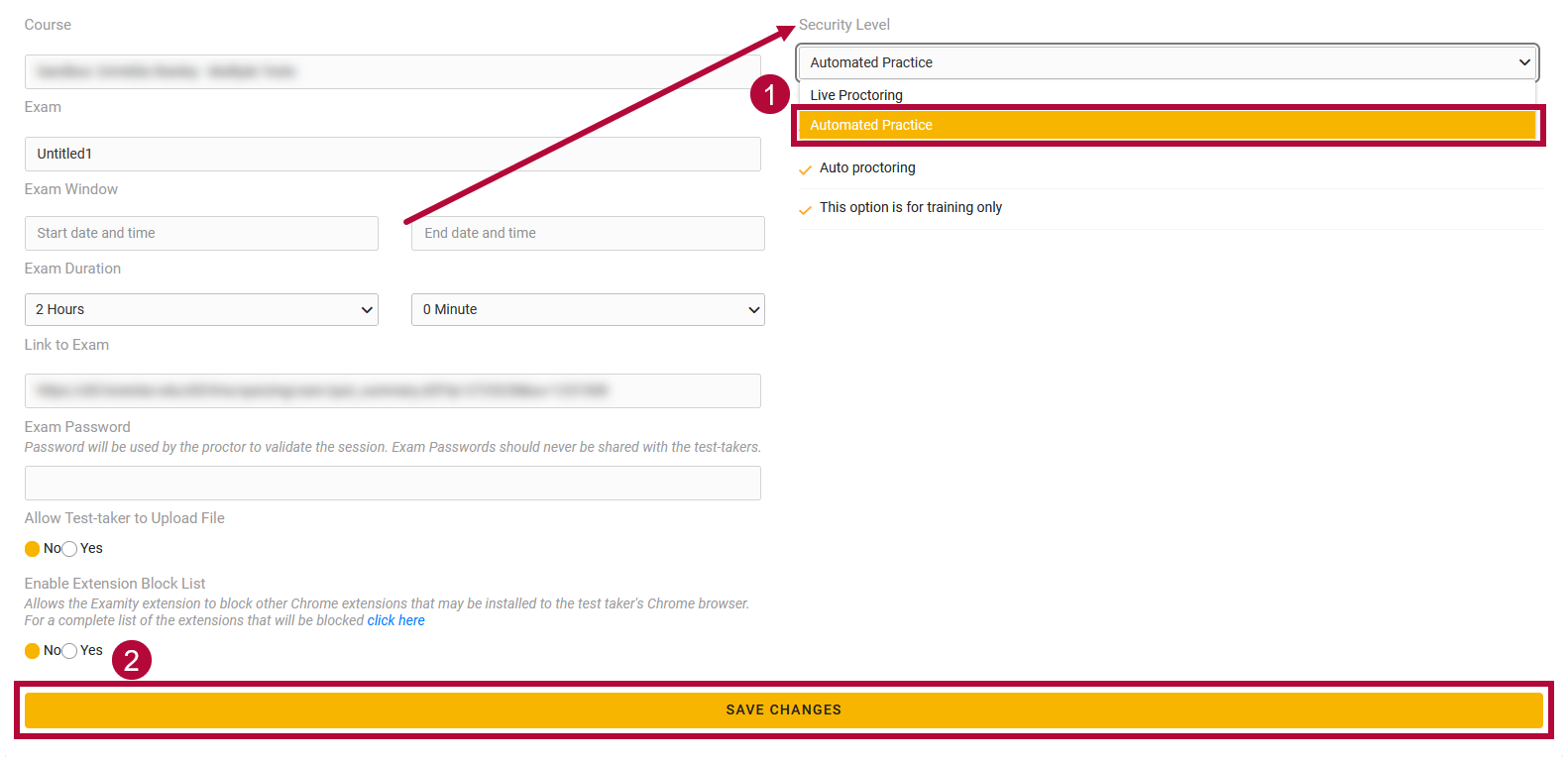The image features a white background with various interface elements related to setting up an online exam. On the left side, a series of options are presented for configuring the exam details. At the top, there is an input field, though the text is blurred out, likely designated for the course name or identifier. Below this field is the label "Exam" followed by "Untitled 1", with "1" being a number that suggests this might be the first exam created in the series.

Further down, several settings for the exam window are visible. These include "Start Date and Time" and "End Date and Time", with corresponding fields to input these details, though they are also blurred out. Following this is the "Exam Duration", which is specified to be "2 hours, 0 minutes". Another field, "Link to Exam", is shown but the link itself is blurred.

The image also displays security settings for the exam. Under "Exam Password", a note emphasizes that this password will be used by the proctor to validate the session and that it should never be shared with test-takers. Additional options include "Allow test takers to upload file", with a choice between "No" and "Yes"; the "No" option is currently selected. There is another setting for "Enable extension block list", which has similar options and is also set to "No".

A notable detail is a round burgundy circle containing the number "2", located near the middle of the image. There is also a prominent banner at the bottom of the options that says "Save Changes".

At the very top, the security level settings are discussed. The current mode is indicated to be "Automated Practice", denoted by the number "1". The text clarifies that "Live Proctoring" and "Automated Practice" with "Auto-Proctoring" are selected options, with the latter specifically noted as being for training purposes only.